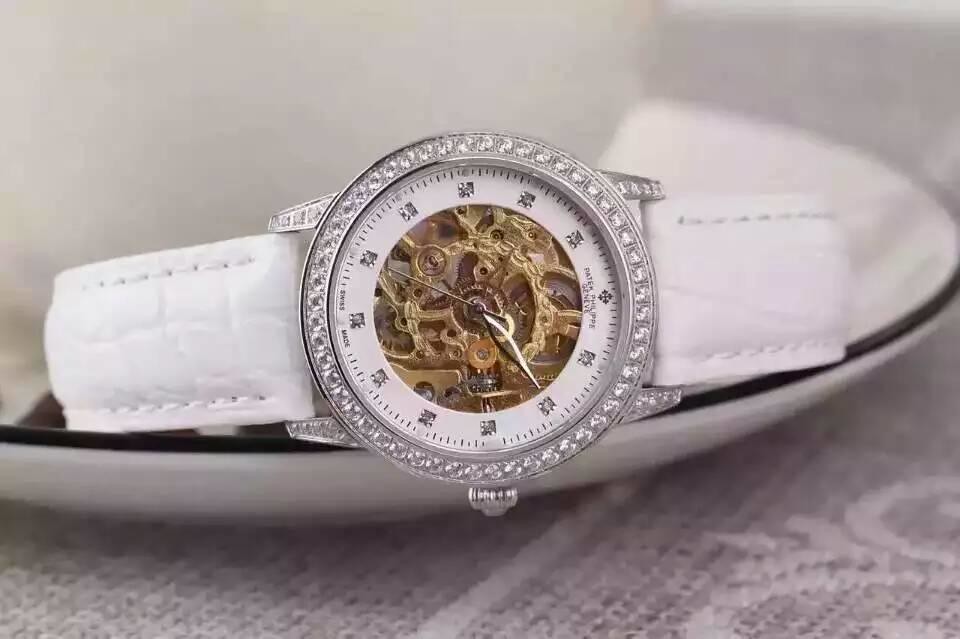This is a close-up photograph of a beautifully detailed wristwatch. The watch is displayed on a lace tablecloth with intricate embroidery, giving it a soft and delicate background. The watch itself rests in an elegant white jewelry holder with a black rim. It features a white leather band that mimics the texture of alligator or snakeskin. The watch face is adorned with a border of what appear to be diamond studs, which also form the numbers around the face. The inner part of the watch face reveals its sophisticated, gold inner mechanisms, showcasing the intricate gears and spinning pieces. The timepiece's hands and winding knob are also gold, adding a touch of luxury to the overall design. The watch is positioned with the knob facing downwards, creating a captivating and detailed visual.